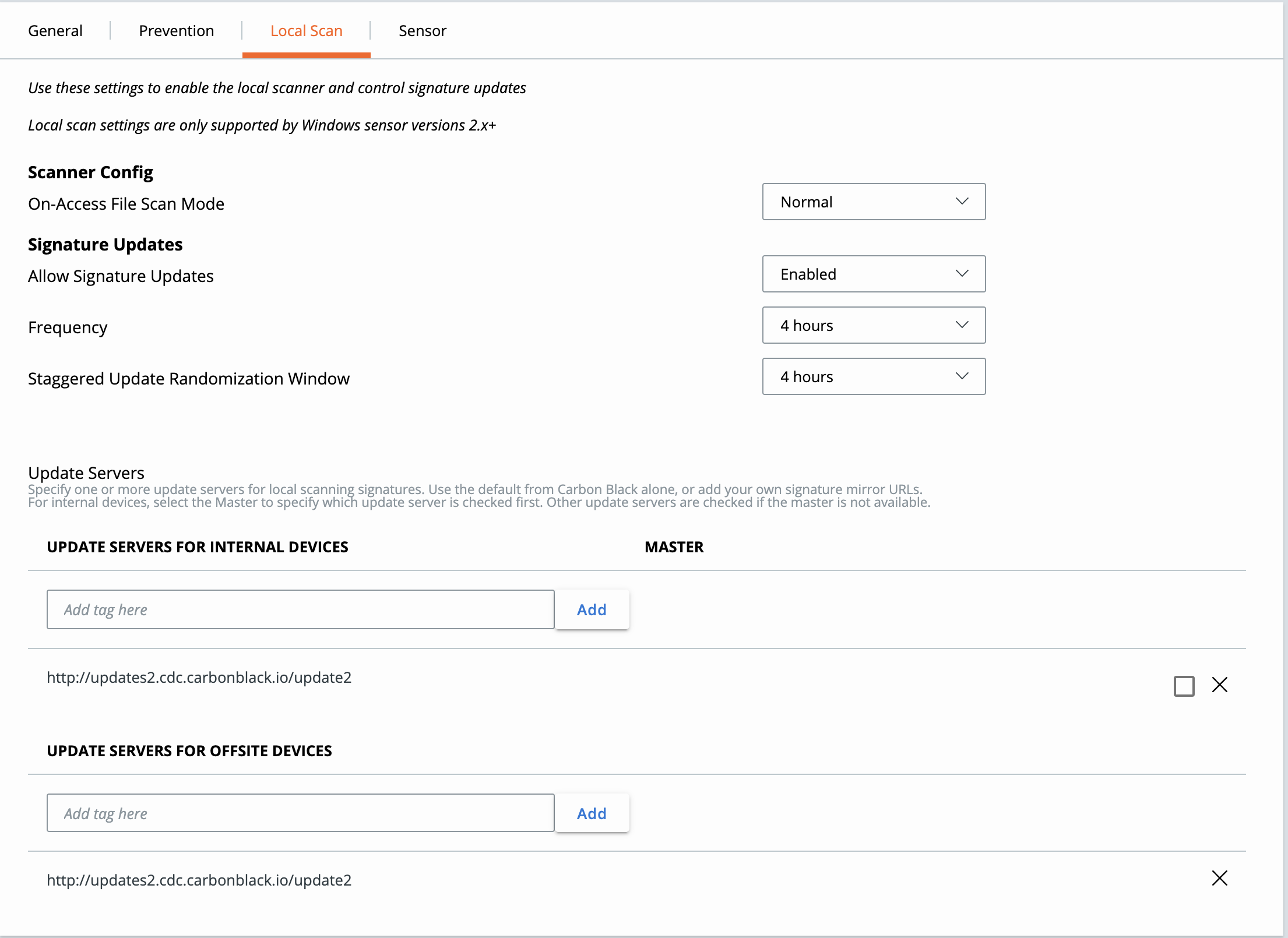**Caption:**

The image displays a configuration page for server and scanner settings. The top section features a navigation menu with options labeled as "General," "Prevention," "Local Scan," and "Sensor." The "Local Scan" option is highlighted with an orange underline.

The main title on the page reads, "Use these settings to enable the local scanner and control signature updates." Beneath it, a brief note in black text states, "Local scan settings are only supported by Windows Sensor versions 2.x and above."

The configuration section includes:

1. **Scanner Version:** Options to choose the version of the scanner.
2. **On-Axis File Scan Mode:** A drop-down menu shown with the selection "Normal."
3. **Signature Updates:**
   - *Allow Signature Updates:* Displays as "Enabled."
   - *Frequency:* Set to "4 hours."
   - *Staggered Update Randomization Window:* Also set to "4 hours."

Below, a section titled "Update Servers" presents instructions for specifying one or more update servers for local scanning signatures. Users can either use the default settings or add their own signature mirror URLs. For internal devices, a "Master" server can be designated to determine which update server is checked first; other servers are only used if the "Master" is unavailable.

Additional fields are provided to input update servers for both internal and off-site devices:
- **Update Servers for Internal Devices:** Includes a field labeled "Master" with an empty input box and a tag saying "Add Tag Here" accompanied by an "Add" button.
- **Update Servers for Off-Site Devices:** Similar to the internal devices section, it includes empty fields and an "Add" button.

Various addresses appear beneath each of these input fields, presumably to indicate sample or existing update server URLs.